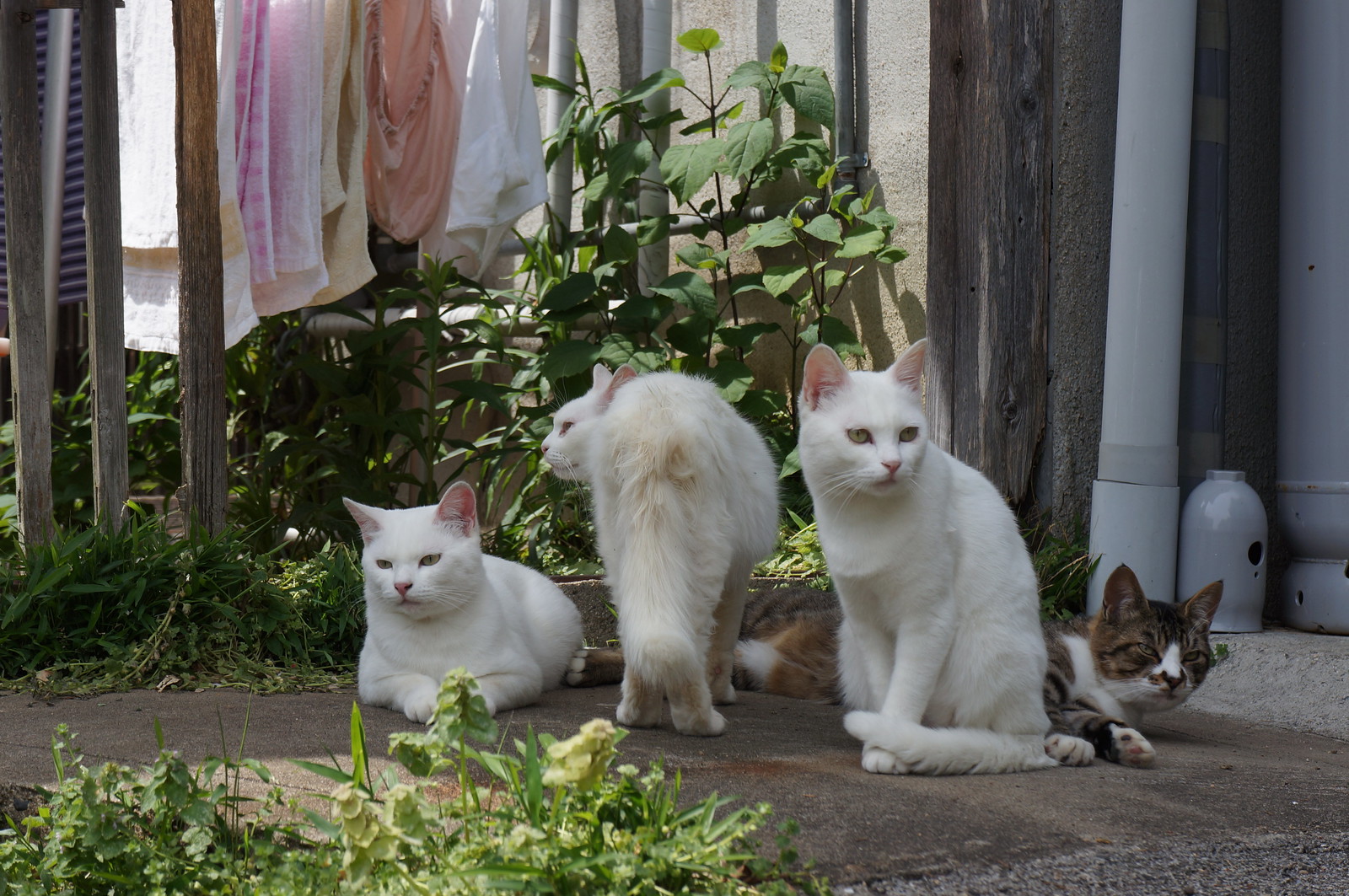The photograph captures a serene outdoor scene featuring four cats on a small patio surrounded by green plants and shrubbery, next to an old wooden fence with laundry hanging in the background. From left to right, the first cat is a white cat lounging sphinx-like on its stomach, facing forward but gazing into the distance to the left. The second white cat is standing, its body facing away from the camera with its left side profile and curled tail in view. The third white cat is seated, looking off to the lower right side of the frame. The last cat, a striking mix of tabby colors—brown, black, and white—lays on its left side with its head perked up, peeking behind the seated white cat. The image, seemingly captured from a low or ground-level perspective, suggests a peaceful scene of pets lounging contentedly on a sunlit patio.